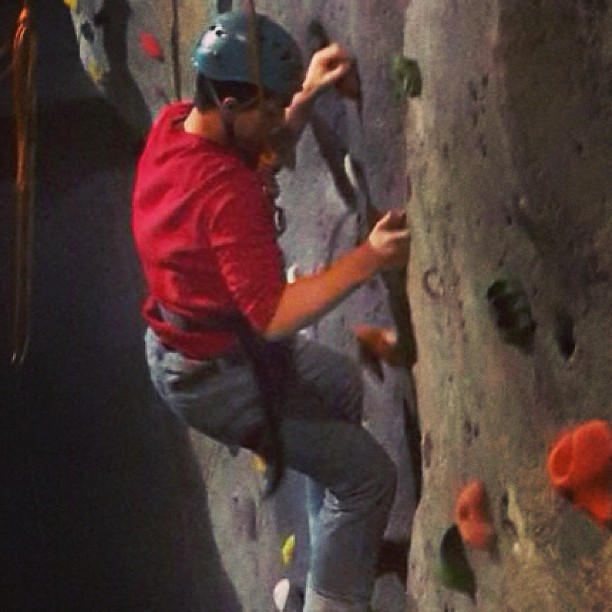The photograph, which is square in shape, captures a young man engaged in indoor rock climbing. He is dressed in blue jeans and a red shirt, with the sleeves pushed up to his elbows, and wears a blue helmet for safety. The man is secured with a harness around his waist, indicative of the protective gear typically used in such activities. The climbing wall he is ascending is located within a recreational facility, characterized by its artificial design. Various brightly colored footholds and grips—red, orange, yellow, green, and white—are embedded in the tan-colored rock wall, aiding climbers in their ascent. The overall image has a soft focus, creating a slightly dreamy effect, though not entirely sharp.